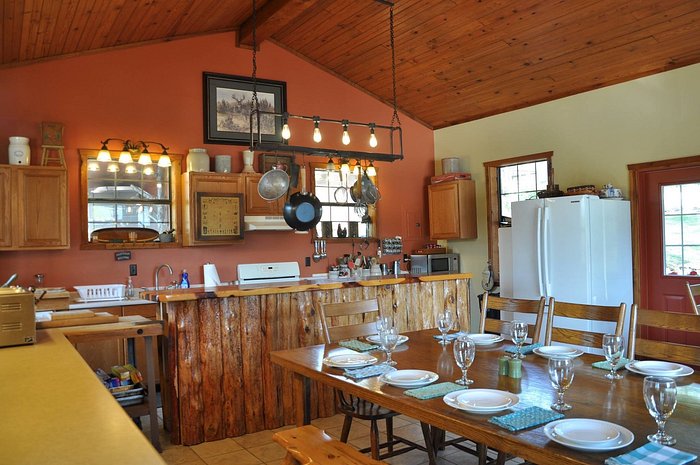The image showcases a spacious kitchen and dining room area with a warm, inviting atmosphere. Dominating the scene is a long, brown wooden dining table meticulously set with shiny white ceramic plates, clear glass cups, and an assortment of green, blue, and blue-green napkins. Surrounding the table are matching brown wooden chairs, and a pair of benches add a rustic charm. Above, a wooden-colored ceiling with hanging yellow light bulbs bathes the room in a cozy glow, enhancing the wood cabinetry that spans the kitchen. To the right of the table, the kitchen counter stands, its mustard-colored surface clean and orderly, with a white refrigerator positioned against the far-right wall. The kitchen area is well-organized, featuring hanging pots and pans, a microwave on one corner of the counter, and a sink with a faucet right behind. The overall ambiance is one of tidiness and warmth, providing a comfortable setting for both cooking and dining.